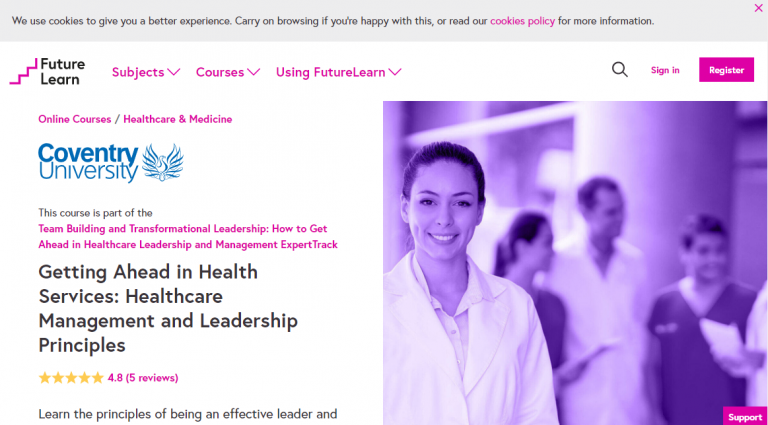### Detailed Caption

The image is a screenshot of a Coventry University webpage hosted on the FutureLearn platform. The page has a sleek, professional design with a white background. At the very top of the image, there is a gray banner displaying a message in a darker gray font: "We use cookies to give you a better experience. Carry on browsing if you're happy with this or read our cookies policy for more information." A pink-colored "X" is located in the upper right-hand corner of this banner for dismissal.

In the upper left-hand corner of the website, a pink staircase icon is placed next to black text that says "FutureLearn." Adjacent to this are pink text links labeled "Subjects," "Courses," and "Using FutureLearn," each with drop-down menus for further navigation. A search bar and buttons for "Sign in" and "Register" are located on the upper right-hand side of the page.

The main section of the webpage is focused on an online course categorized under "Healthcare and Medicine" offered by Coventry University. The Coventry University logo features prominently in blue, with an emblem that resembles a phoenix or peacock. The course title is part of the "Team Building and Transformational Leadership" track, specifically labeled "How to get ahead in healthcare leadership and management expert track." The course description includes "Getting ahead in health services, healthcare management and leadership principles."

The rating for this course is displayed as a 4.8 out of 5 stars, based on five reviews. Although the course description starts with "Learn the principles of being an effective leader," it gets cut off, leaving the full text unreadable.

To the right of the course information, there is a visually appealing purple-toned image featuring a young woman in a lab coat. She stands smiling confidently, surrounded by colleagues, illustrating a collaborative and professional healthcare environment.